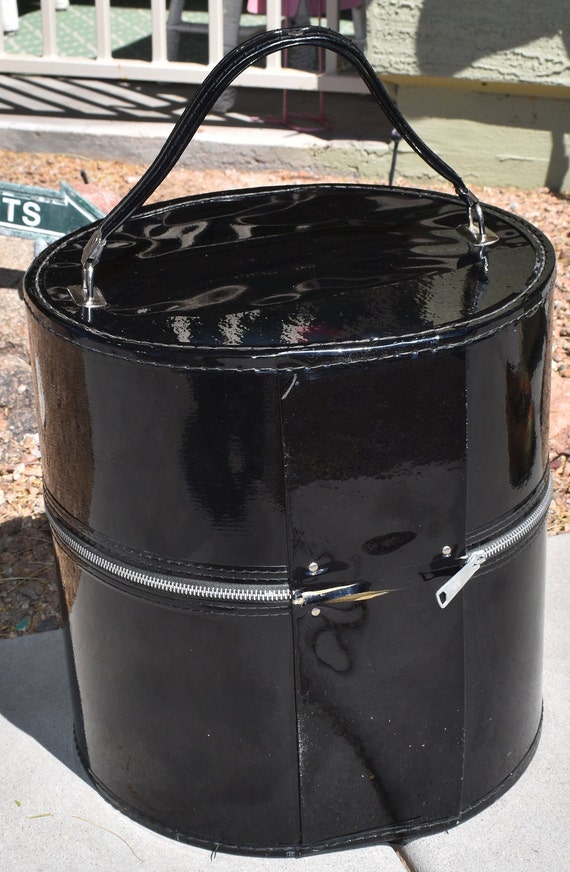The image depicts a close-up of a tall, round, black carrying case, reminiscent of a drum or hat box, made from a shiny vinyl material. The case features a handle on top with silver trim and a zipper that extends around its middle, allowing it to open into two cylindrical halves. The threading appears worn, suggesting some age. It is photographed outside on a gray concrete sidewalk, with mulch and foliage visible in the background, and a portion of a green house, adding depth to the scene. A small white fence and a stone or concrete wall are also discernible in the upper part of the image, hinting at a yard sale setting.